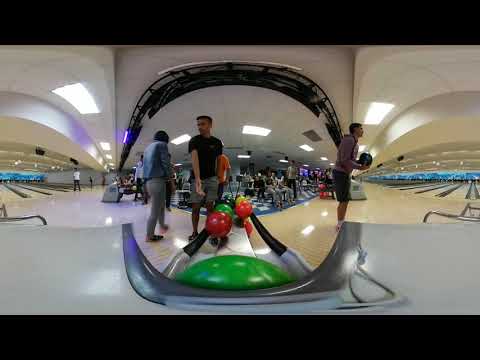The image is a 360-degree view of a bustling, spacious bowling alley with high ceilings and fluorescent lights. In the center, above a ball return, someone in a black t-shirt and shorts is about to pick up a red bowling ball. Around the ball return are several brightly colored bowling balls, including two green, two red, and a yellow one. To the side, a person wearing long pants and a jean jacket stands nearby. On either side of the ball return, there are about a dozen tan-colored lanes, with blue tops, visible, where a person in a purple sweater and black shorts is holding a blue bowling ball, deciding which lane to approach. The background shows blue and white tile flooring leading to a seating area and a concession stand, with approximately 20 to 30 people, although they appear small and their clothing details are indistinguishable. The scene captures a lively atmosphere of families and friends enjoying a fun day of bowling.